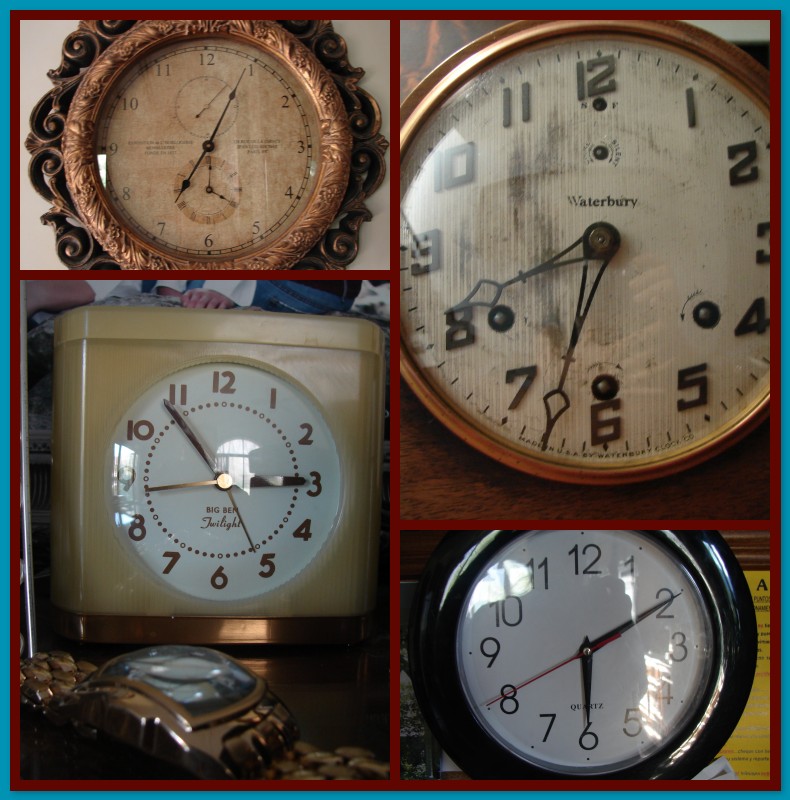The image is a color photo collage of four distinct wall clocks, framed by a blue border with an inner red border. Each clock is presented in a separate panel, divided by red lines. 

- In the top left panel, there's an antique wall-hanging clock featuring an aged white face with black numerals and hands. This clock also includes a smaller additional clock and has a gold-colored frame.
- The top right panel shows a clock with a smudged white face, black hands, and numerals encased in a copper-colored frame. This clock is marked with the word "Waterbearing."
- In the bottom left panel, there is a rectanglar-shaped clock that resembles an oiler base, with a white face and brown numbers. The clock includes black and gold hands for hours, minutes, and seconds.
- The bottom right panel displays a sleek, black plastic round clock with a white face, black hands, black numerals, and a distinct red second hand. It is labeled "Courts of the Six."

In addition, there's a partially visible gold wristwatch in the bottom left corner, although its face isn't completely visible. Each clock brings a unique design element to the collage, ranging from antique to modern styles.